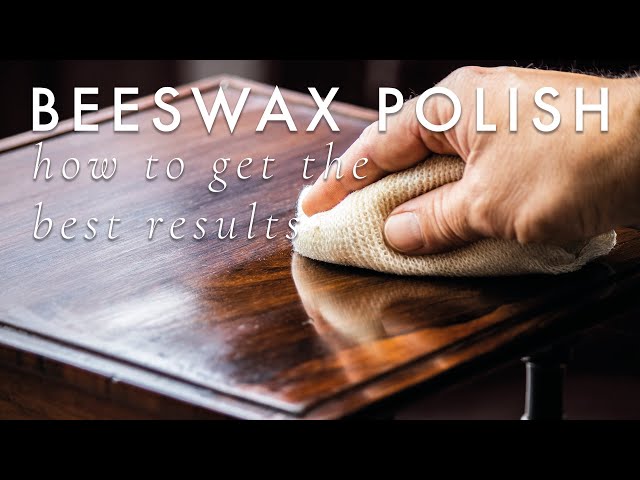In the center of the horizontally aligned rectangular image, a man's right hand holds a tan, textured polishing cloth, resembling cheesecloth, and diligently wipes the surface of a small, high-end, square wooden table. The portion of the tabletop being polished is noticeably shinier and free of dust, creating a stark contrast with the still dusty, blurred back section. The tabletop exhibits rich, dark wood grains that add to its elegant appearance. Overlaying this scene, white text is prominently displayed against black letterbox borders at the top and bottom of the image. The text reads, in a mix of capital and lowercase letters: "Bees Wax Polish - How to Get the Best Results." The overall composition and prominence of the text suggest the image might be an advertisement for Bees Wax Polish, emphasizing the product's effective results against the dark backdrop, making the polished shine of the wood stand out.